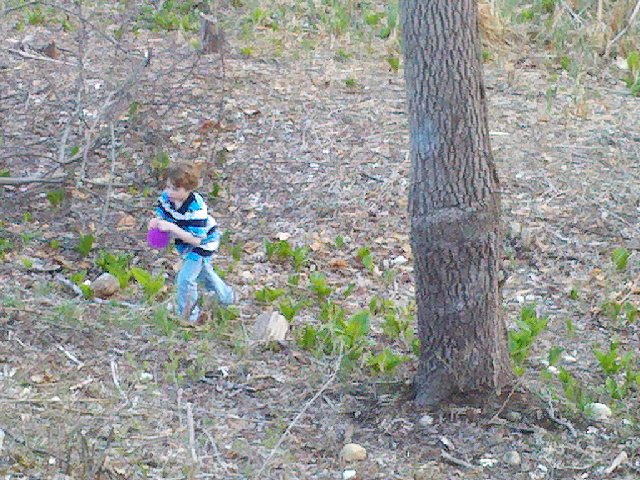In the photograph, a young boy, approximately seven years old with brownish-reddish hair, is captured walking through a forest during what appears to be the fall season. He is the sole subject of the image, positioned centrally amidst a natural setting filled with sticks, rocks, and fallen brown leaves scattered across the flat, earthy ground. The scene is punctuated with patches of green grass and foliage sprouting here and there. The boy is dressed in a navy blue shirt featuring powder blue and white stripes, paired with long light blue jeans. In his hands, he holds a purple object, which could be a ball or a bag. To the right of the boy stands a tall tree, its trunk extending out of the frame. Another tree is visible in the background, contributing to the forested atmosphere. The photograph is devoid of any text or date markers and is likely taken in a backyard, hill, or secluded natural area, possibly during a family hike or outing. The overall color palette of the image includes shades of tan, brown, green, light blue, purple, black, orange, and gray, suggesting a midday setting.